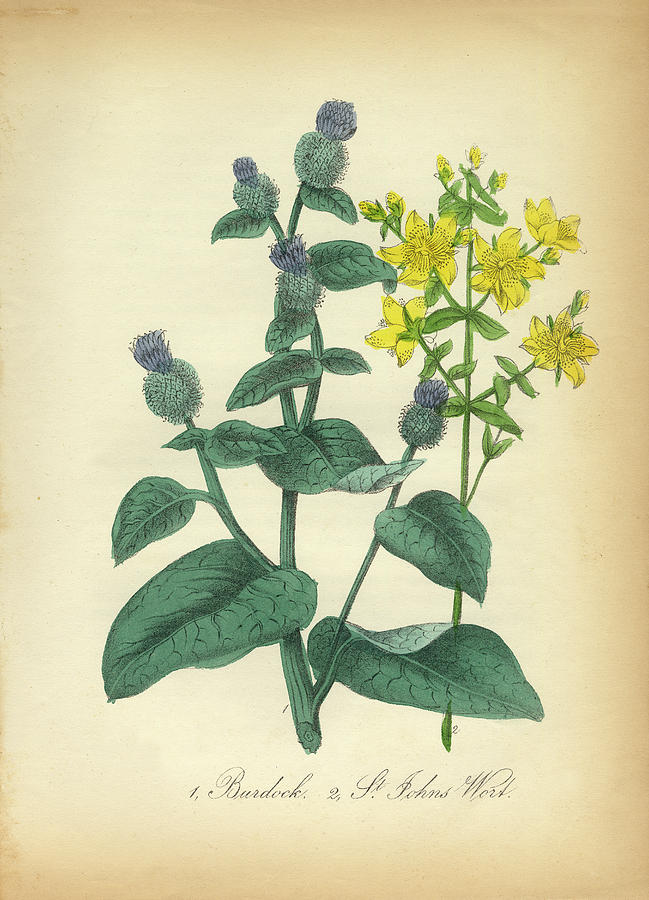The image depicts a full-color drawing on what seems to be aged, beige paper with darker edges and a cream-colored center. The artistic rendering features two distinct plants. The plant on the left has a prominent large green stem with several offshoots, each adorned with large, textured green leaves. At the tops of these stems, green buds are visible, partially unfurling to reveal small blue petals that peek out. To the right, a different plant with a slimmer, lighter green stem and smaller leaves is depicted. This plant features bright yellow, star-shaped flowers with pointed petals and a central pollen spike. Each of these flowers has approximately five to six petals. Beneath the illustration, written in cursive, are labels identifying the plants as "1. Burdock" and "2. St. John's Wort."